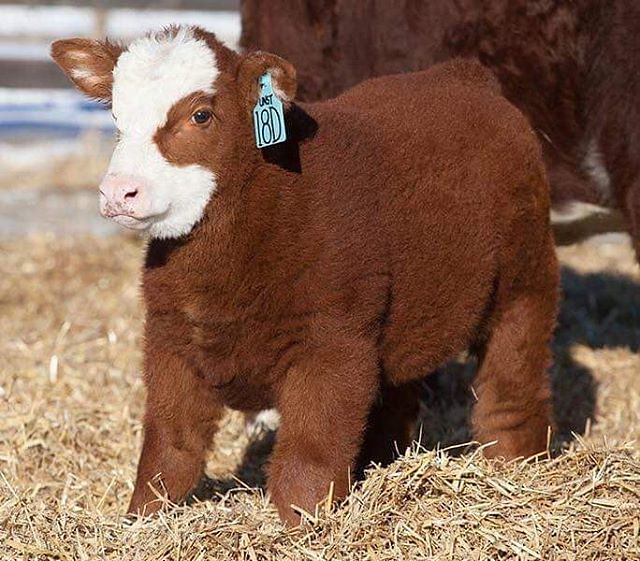This is a color photograph showcasing a close-up of a young calf. The calf stands on all four legs in yellow straw, facing almost directly forward towards the bottom left corner of the image. Its fur is a deep chestnut reddish-brown, with a distinctive white forehead, nose, and chin. The snout is a light brownish-pink, nestled in the white area. The calf has a stocky build and its ears stick straight out, each furry and adding to its thick, soft appearance. A blue tag on its left ear displays the markings "18D" and additional unreadable text above. In the upper right corner, a darker brown adult cow, possibly the mother, appears partially cropped from the photo, adding a sense of scale to the young calf. The backdrop includes grey fencing and blurred blue and white lines, contributing to the scene's farm setting ambiance.